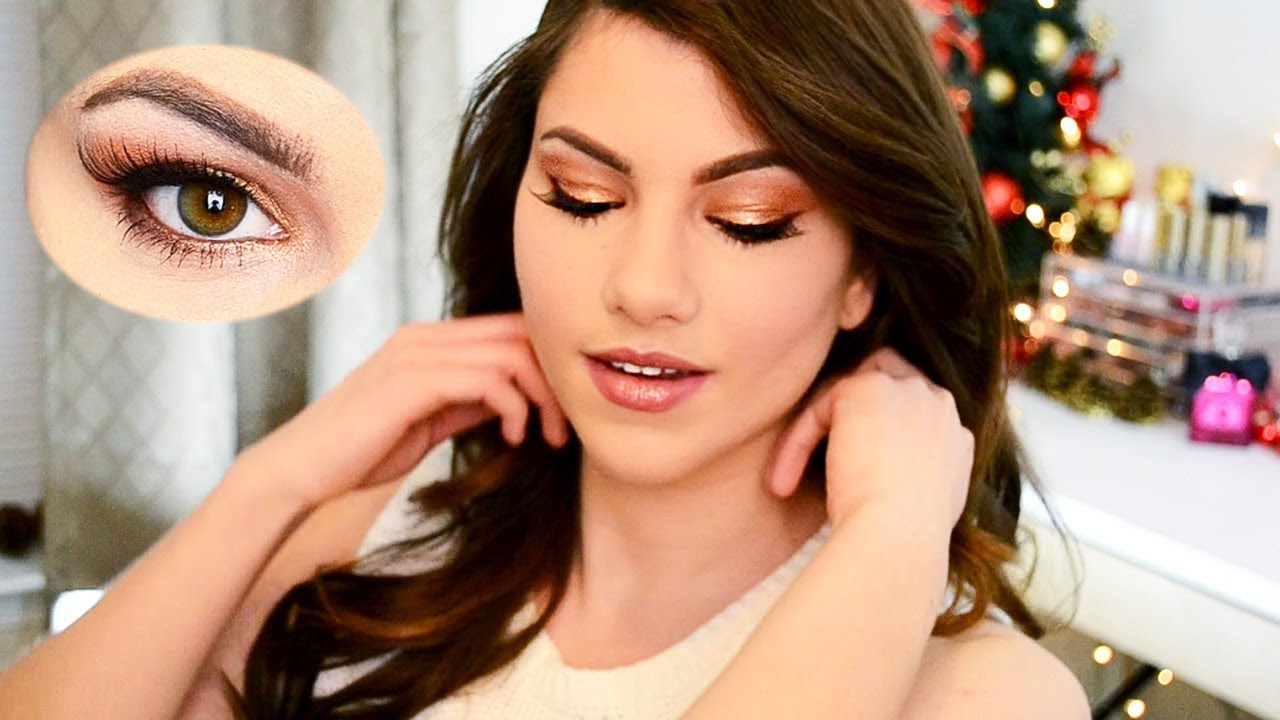The image depicts a close-up of a light-skinned woman with long, dark hair and striking makeup. Her eyes are closed, showcasing her long eyelashes and the intricate green, sparkly brown, and gold eyeshadow. She wears pinkish lipstick and a cream-colored tank top. Her hands frame her face near her ears, as if she's about to flick her hair back. In the top left corner of the main image, there's an oval inset displaying a close-up of her brown eye, highlighting the same elaborate makeup. The background includes a white curtain, a white desk cluttered with various makeup items, and sparkly decorative lights that might be on a Christmas tree. The setting is well-lit, making all the details of her appearance and surroundings vivid and clear.